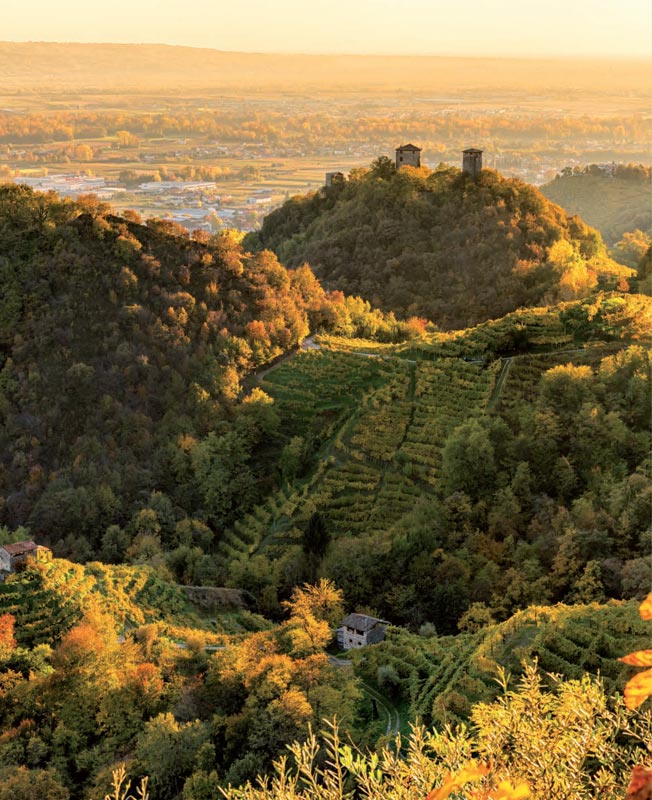This picturesque landscape photo, likely taken in Europe, features a sun-drenched valley nestled between rolling hills and rugged cliffs, captured during the transition from late summer to early fall. The vibrant yet slightly yellowing greenery hints at the changing seasons. Amidst the lush environment, small white houses are scattered, some nestled among various shades of green trees and others perched on the hills, forming a charming patchwork of civilization. The terrain reveals meticulously maintained fields, possibly vineyards or farmlands, with evenly spaced rows suggesting well-tended agricultural activity. Dirt roads crisscross the landscape, winding past tiny shacks and leading up to the hilltops, connecting the isolated homes. Beyond these hills, the distant flatlands and softly glowing morning sunlight create an orangish-red hue, enhancing the serene beauty of this possibly European countryside. The backdrop features a sand-colored mountain range, contrasting against the greenery and adding depth to this captivating aerial photograph.